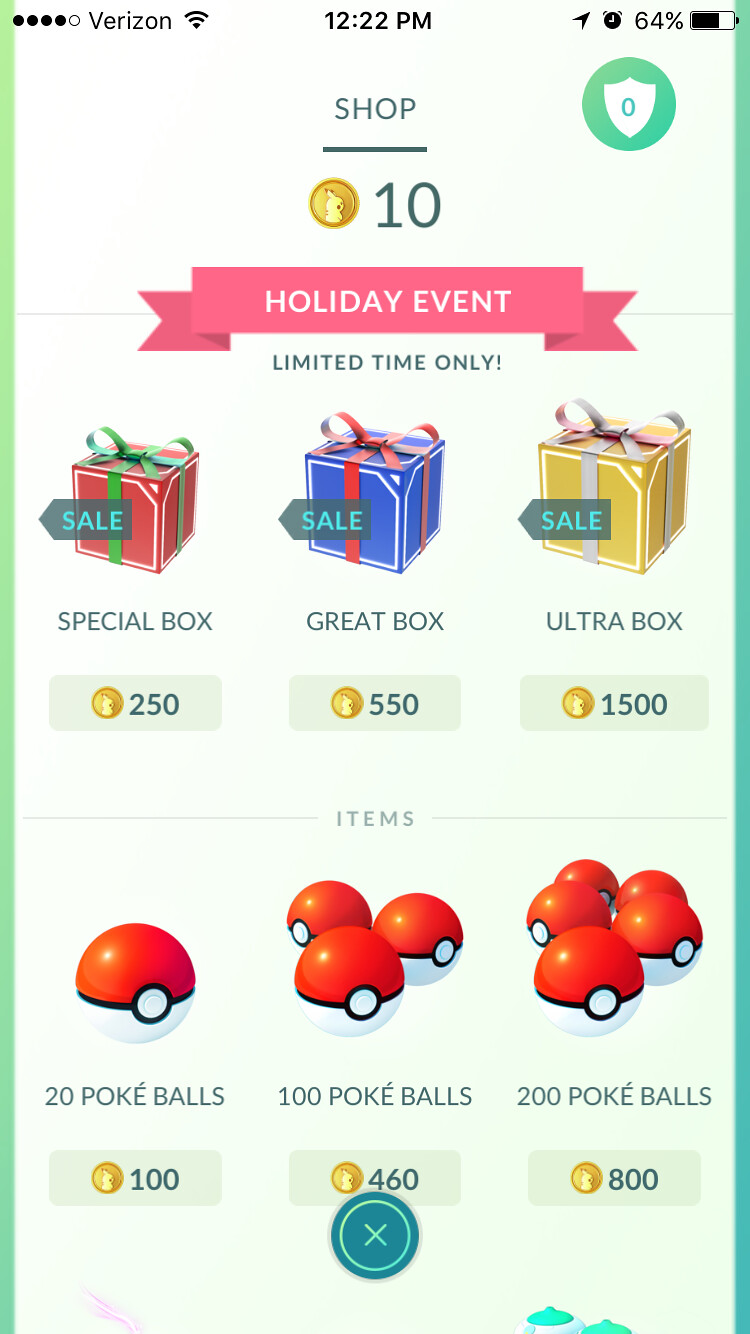This image is a detailed screenshot from the mobile game Pokémon Go, taken on a phone. At the top, the status bar displays "Verizon," a Wi-Fi signal, the time "12:22 PM," and a battery level of 64%. The main screen shows the "Shop" area of Pokémon Go, highlighted by a "Holiday Event" banner in red with white text, indicating a limited-time event. 

Below the banner, there are three colorful boxes tied with ribbons: a red "Special Box" priced at 250 coins, a blue "Great Box" priced at 550 coins, and a yellow "Ultra Box" priced at 1500 coins. Each box prominently displays the word "Sale." 

Further down, the screen offers Pokémon-themed currency options illustrated by pokeballs. These options include 20 Poké Balls for 100 coins, 100 Poké Balls for 460 coins, and 200 Poké Balls for 800 coins. Each option is visually represented by corresponding images of one, three, and six Poké Balls respectively. The presentation clearly indicates the festive, in-game shopping experience tailored for a holiday event.